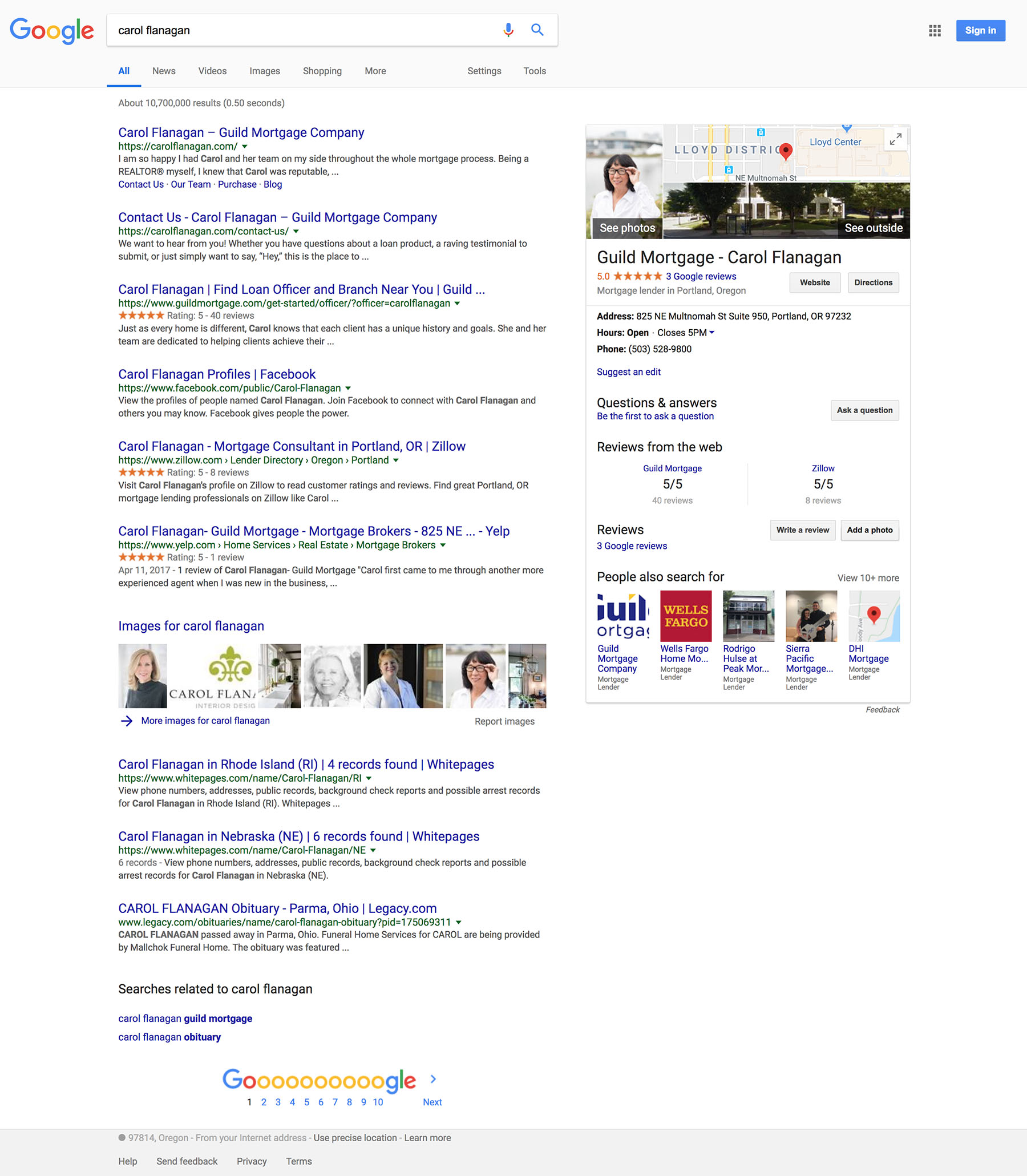The image depicts a Google search results page for "Carol Flanagan." In the top left corner, the iconic Google logo is displayed in its classic blue, red, yellow, and green colors. The search query "Carol Flanagan" appears in the search bar at the center of the page, yielding numerous results about a person named Carol Flanagan associated with the mortgage industry.

The results prominently feature links related to Carol Flanagan at the Guild Mortgage Company, including contact information and details about her role as a loan officer and mortgage consultant in Portland, Oregon. Additional listings include various profiles on social media platforms like Facebook, professional profiles, and even an obituary for someone with the same name.

On the right side of the page, a knowledge panel provides a succinct summary of Carol Flanagan's professional information at Guild Mortgage Company, complete with a photo, office location, and a brief snippet about her positive five-star reviews. The panel also displays additional contact details, including her address and phone number, and suggests other related mortgage companies in the "People also search for" section. The page is packed with information, images, and various clickable links for further exploration.